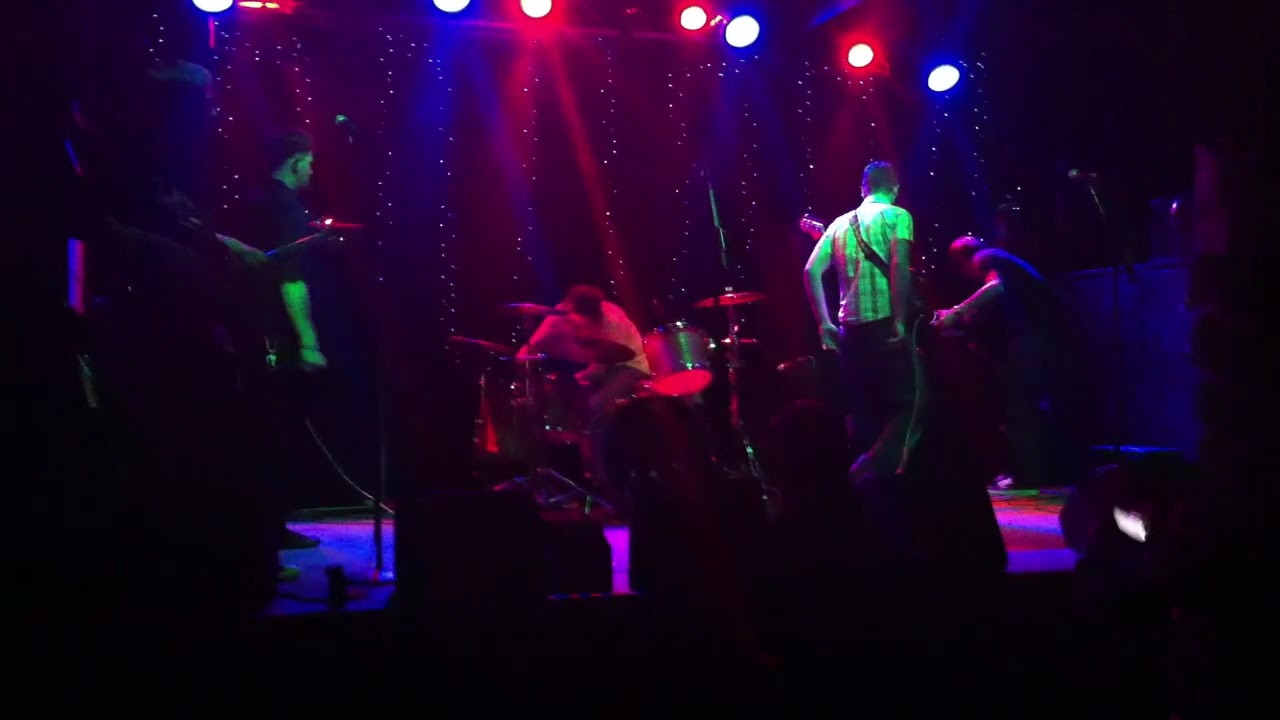The image captures a vibrant and dynamic scene of a concert stage, featuring a five-member band caught in a moment either preparing to perform or post-performance. Dominating the scene, blue and red lights alternate from the overhead rigs, casting a colorful glow on the stage. The drummer, positioned at the back, is illuminated with a red hue, distinguishing him from the others with his lighter shirt. The remaining band members are mostly dressed in dark attire, except for one man prominently wearing a yellow fluorescent shirt and checkered dress shirt, with a guitar strapped to him and his hand in his back pocket as he faces away from the camera. Another member on the right appears to be interacting with something or someone in the corner, adding to the scene's bustle. The background features a starry pattern with small dots of light, contributing to the overall atmosphere. Although the audience is mostly obscured in shadows, a couple of heads can be seen in the foreground, with one person possibly holding a smartphone. This closely-framed shot, likely taken from the front row, focuses intently on the band and the illuminated stage setup.